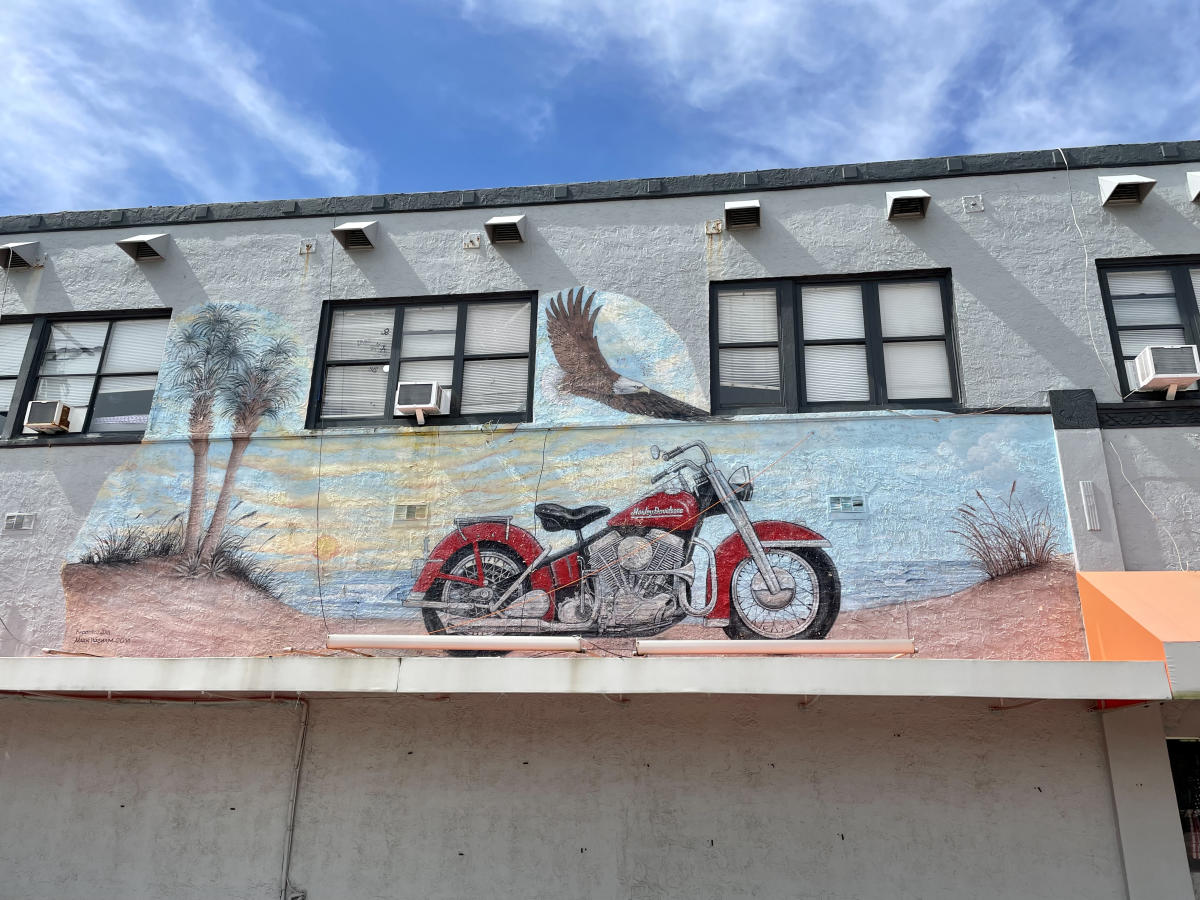This image depicts a vibrant mural painted on the side of a two-story concrete building. The mural, which spans from the first story up to the second story roofline, captures a picturesque beach scene. At its center, a red Harley-Davidson motorcycle with chrome accents sits prominently on the sand. Surrounding the motorcycle, the mural features two tall palm trees and a bald eagle soaring overhead against a clear, blue sky. The backdrop is alive with waves crashing onto the shore and scattered clouds dotting a sunlit sky. The building itself appears to be multi-use, with multiple windows, each equipped with air conditioning units and blinds. The bottom section of the building has a main entrance on the right side, but is otherwise plain compared to the richly detailed mural above. The actual sky above the building mirrors the mural with its blue expanse and misty white clouds, suggesting the photo was taken during the day.